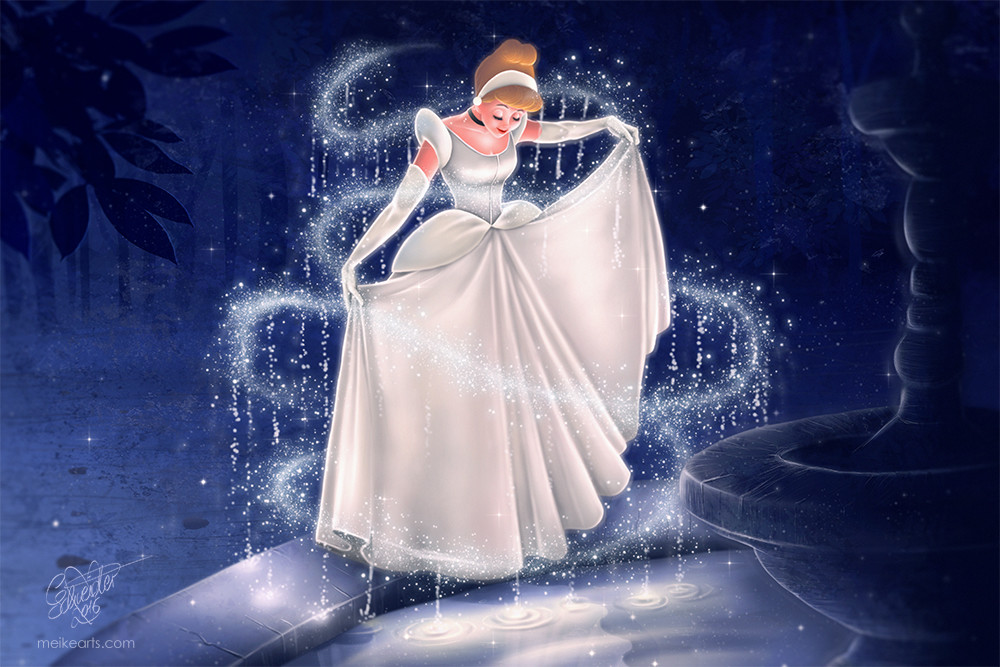This image, presumably from the film "Cinderella" or created in the distinctive style of Disney's classic, showcases the iconic moment when Cinderella first dons her magical white gown. The scene is set at nighttime near an elegant fountain, where Cinderella, with her hair in a graceful bun adorned by a silver headband, is lifting the sides of her shimmering silver-white dress, as tendrils of golden and white sparkles weave around her. Her outfit is meticulously detailed with puff sleeves, a fitted bodice, and a long flowing skirt. She complements her dress with long matching gloves, a black choker, and earrings. Cinderella gazes into her reflection, the swirls of magic enhancing the ethereal quality of this transformative moment. The unique illustration style is credited to mykeekaarts.com, capturing the fairy tale essence perfectly even if Cinderella’s facial features deviate slightly from the classic Disney depiction.